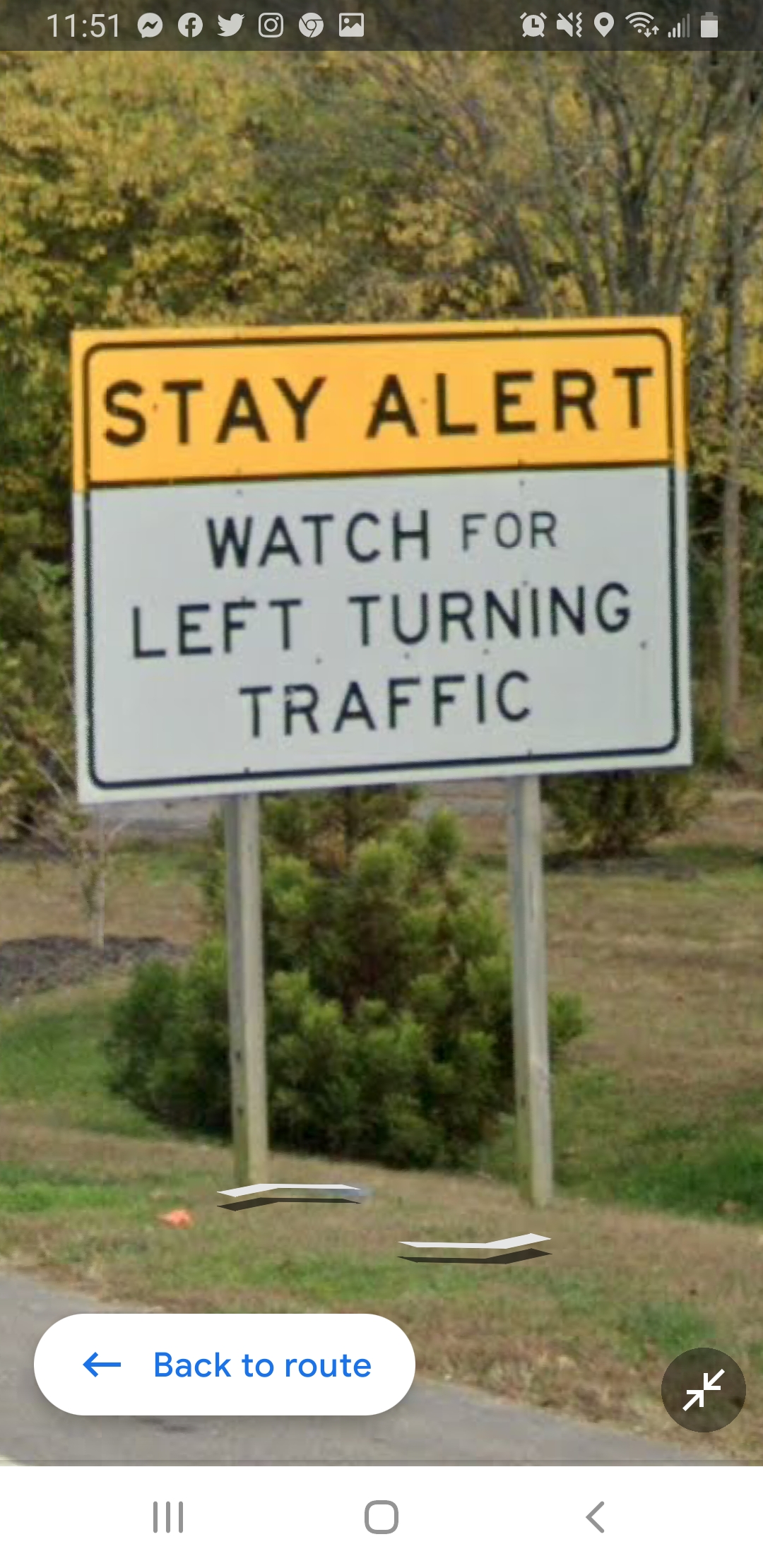The image is a screenshot taken on a smartphone, displaying a scene from Google Maps or Google Earth. At the top of the screen, the phone's status bar shows it is 11:51 AM and includes icons for Messenger, Facebook, Twitter, Instagram, photos, Wi-Fi signal, battery life, and three signal bars. At the bottom left corner, there's a pill-shaped white block with blue text and an arrow pointing left, stating "back to route."

In the image itself, prominently positioned on the side of a road, there's a traffic sign. The sign, mounted on two poles, has a bright yellow-orange background with bold black lettering that reads "Stay Alert," and below that, in a grey block with black lettering, it says "Watch for left-turning traffic." The setting includes a grassy area with a small shrubby tree immediately behind the sign and larger trees with leaves changing color in the background. Additionally, the edge of the road and more greenery are visible at the bottom of the scene.